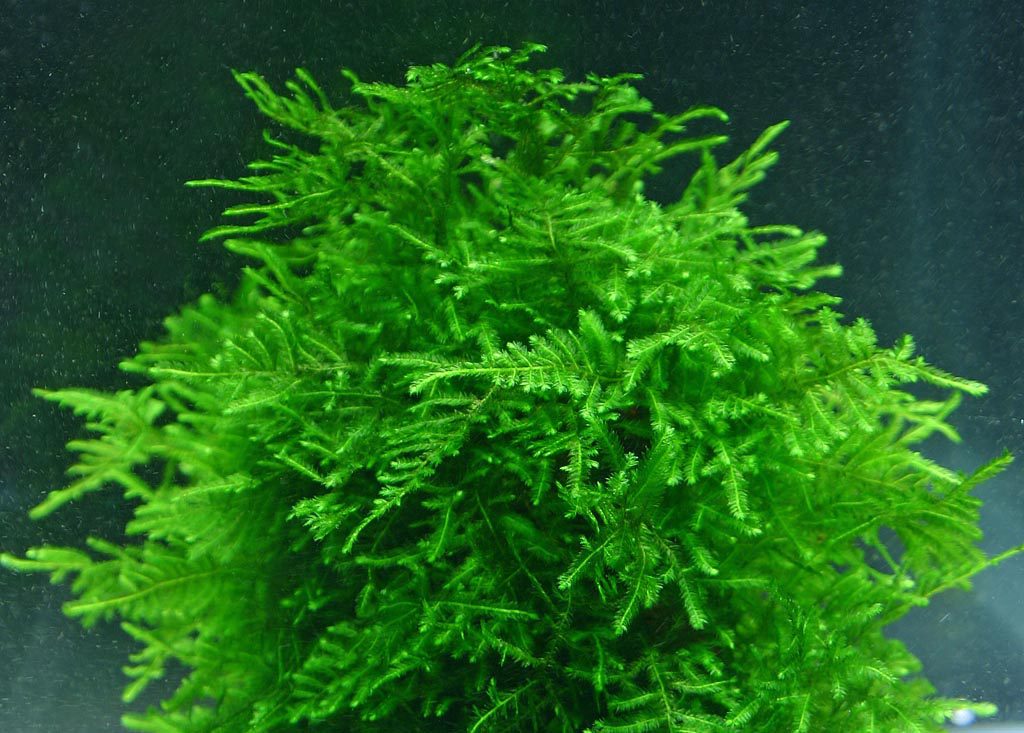This detailed photo showcases a vibrant green aquatic plant species, characterized by a large bundle of long, feather-like leaves that exude a soft and slightly pointy appearance. The plant, reminiscent of underwater moss, is positioned within an aquarium environment, as suggested by the dark teal, speckled background and floating particles. The bright green leaves appear almost luminous, giving off a glowing effect under the aquatic light. The plant exudes a lush and thriving presence within its watery habitat, underscoring its likely use in aquarium settings for its aesthetic appeal.